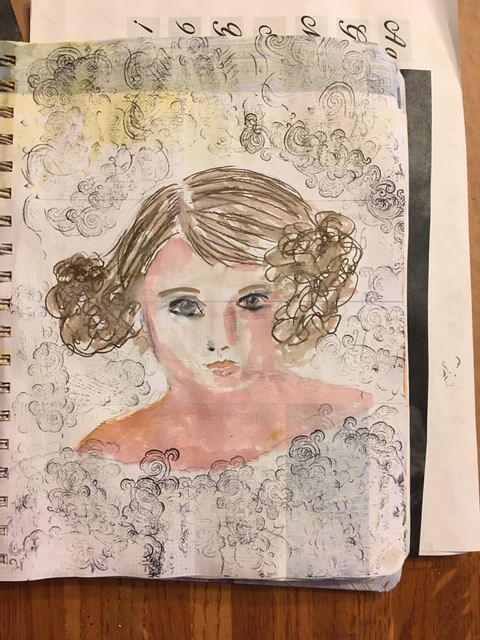This photograph captures a detailed mixed-media drawing of a woman with light pink skin. Her chin-length, curly brown hair frames her face, which features dark eyes, pink lips, and light brown to golden eyebrows. The portrait, rendered in a combination of watercolor, pencil, and marker, focuses on her head down to her collarbone. Surrounding her are intricate, swirling billows of black and white smoke-like patterns, suggestive of misty clouds. The artwork is set against white paper, likely still attached to a spiral-bound sketchbook, with visible binding on the left. In the background, faint cursive words can be seen, adding a subtle textual element to the composition.